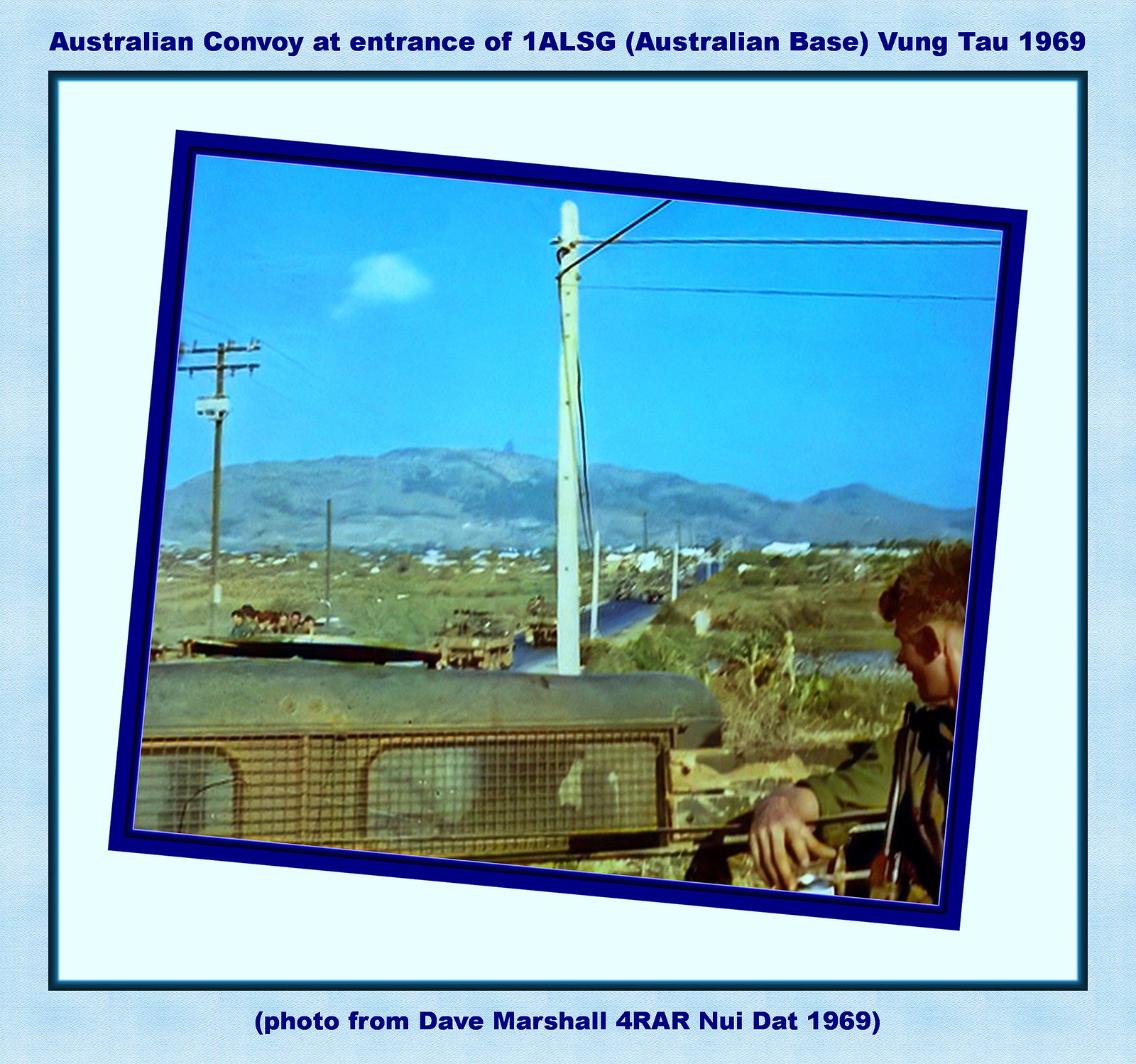The square image features a central photograph slightly tilted with its left side up and right side down. The photo is bordered by a white or light blue background with a black pinstripe and an outer powder blue frame. At the top of the powder blue border, in dark blue print, it reads, "Australian convoy at entrance of 1 ALSG (Australian base) Vung Tau 1969." At the bottom, the caption in blue font states, "(photo from Dave Marshall for RAR Nui Dat 1969)."

The central photograph captures a young Caucasian man, likely in his early 20s, seated in the back of a truck, looking ahead at a convoy of similar military vehicles. These open-back trucks are filled with soldiers and are traveling down a road flanked by power lines and dead trees. In the background, there is a town set against a mountain range with a clear blue sky above. A prominent cloud is visible in the top left corner of the image.